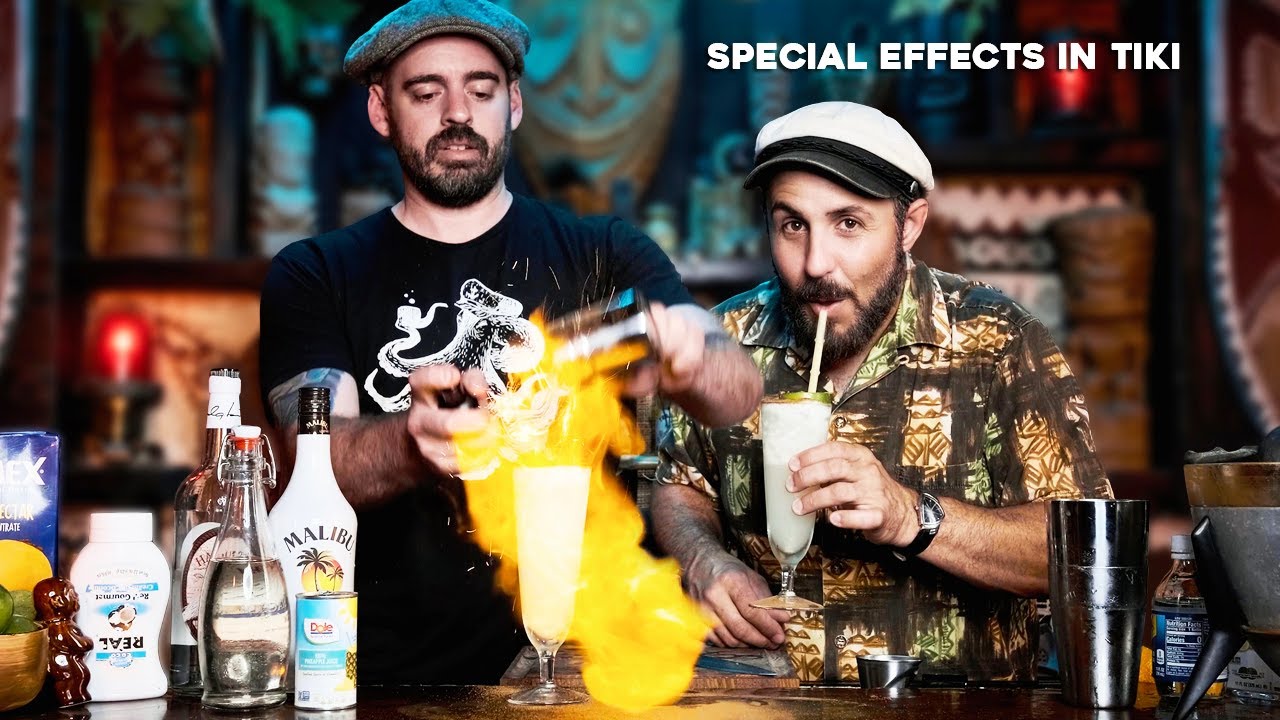The vibrant, full-color photograph captures two bearded men standing behind a well-stocked bar, illuminated by indoor artificial light. The horizontally rectangular image prominently displays a playful text overlay in all caps at the upper center-right: "SPECIAL EFFECTS IN TIKI." 

On the right, a man wearing a detailed brown, tan, and green Hawaiian shirt and a white and black captain's hat is sipping a white cocktail through a straw, his expression mischievous. His cocktail glass contains what appears to be a piña colada. His shirt features tribal patterns, enhancing the Tiki bar atmosphere. Behind him, the bar is adorned with tiki statues and masks, contributing to the exotic ambiance.

To the left stands a slightly taller man in a black short-sleeve shirt adorned with an octopus wearing a sea captain's hat while holding a pipe. Topping off his look is a gray newsboy cap. This man is focused on his task, igniting a concoction, with flames dramatically leaping up from the bar as he presumably mixes a flaming drink. Surrounding them on the bar are various bottles of alcohol, including coconut rum and pineapple juice, essential ingredients for crafting tiki cocktails.

The combined details of the men's attire, their actions, and the captivating bar setup create an engaging snapshot, seemingly a thumbnail for a lively YouTube video exploring tiki-themed special effects.